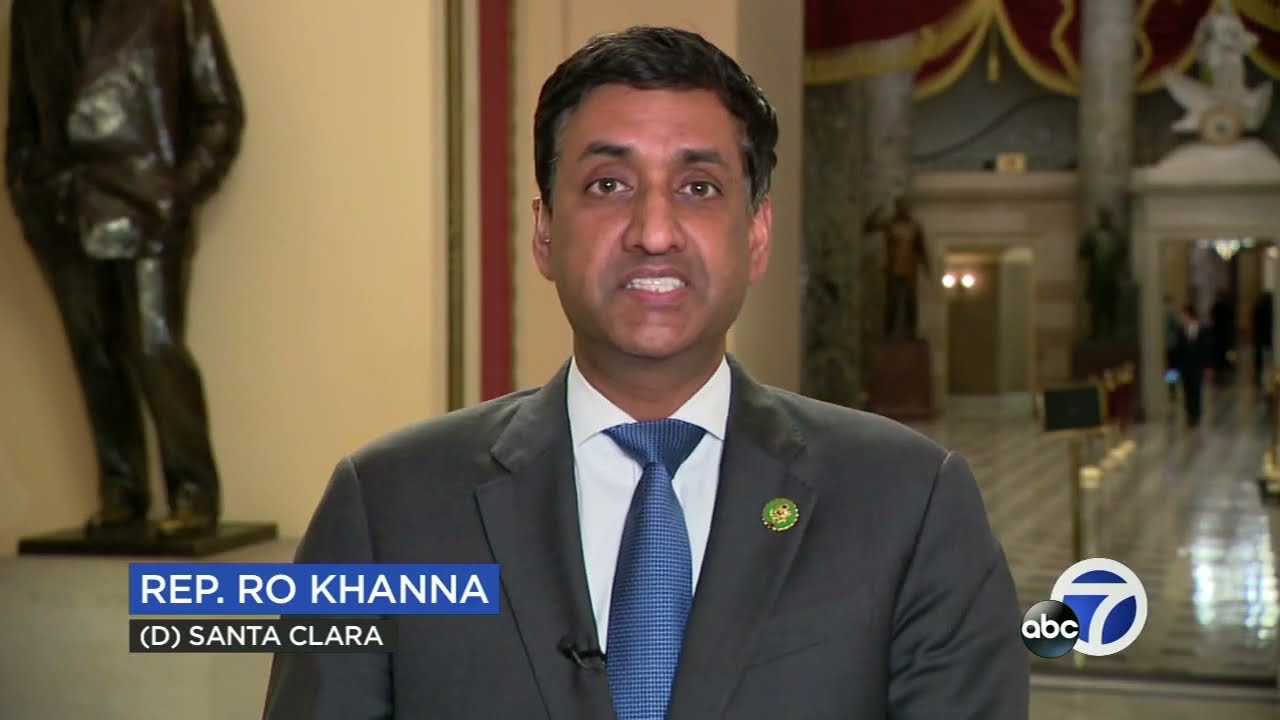This is a screen grab from what appears to be a local ABC News broadcast, indicated by the ABC logo overlaid on a Channel 7 logo situated at the lower left of the image. The text on the screen displays "Rep. Ro Khanna" in white against a blue background, and "D, Santa Clara" in white against a black background, identifying the individual as Representative Ro Khanna, a Democrat from Santa Clara.

The focal point of the image is Representative Ro Khanna, who is directly addressing the camera. He is dressed in a gray suit, a blue tie, and a white button-down shirt, and he is wearing a green pin on his left lapel. Khanna is an Indian-descendant man with neatly combed, short hair. 

The setting appears to be a political building, possibly the House of Representatives or a significant state building in California. Behind him is a bronze statue of a man with his hands in his pockets. The background features white walls with red trim, red curtains, and pillars adorned with other statues, as well as red ropes marking walkways. This image captures Khanna discussing a political matter on this news broadcast.